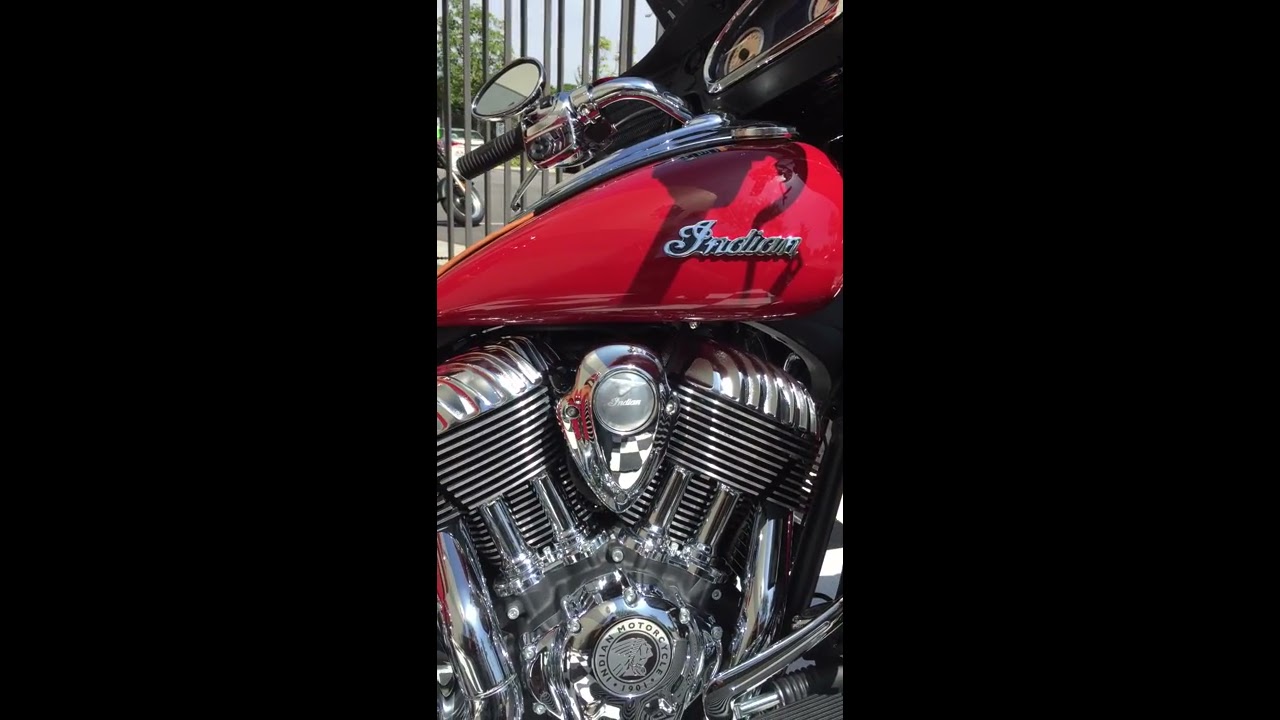The close-up vertical image showcases a beautifully maintained Indian motorcycle, prominently displaying its candy apple red gas tank with chrome "Indian" script. Visible are slight white marks that might be scratches or reflections. The bike features black hand grips on silver handlebars, a circular left side mirror, and the bottom half of a windshield. The slanted chrome gas tank cover and two similarly sized gauges are set below the windshield. The polished chrome engine proudly bears the "Indian Motorcycle 1901" logo with an Indian chief head. Surrounding the central bike image, there are wide black borders, while faintly in the background, a parking space is discernible, possibly with another motorcycle’s wheel and a glimpse of a tree and sky.